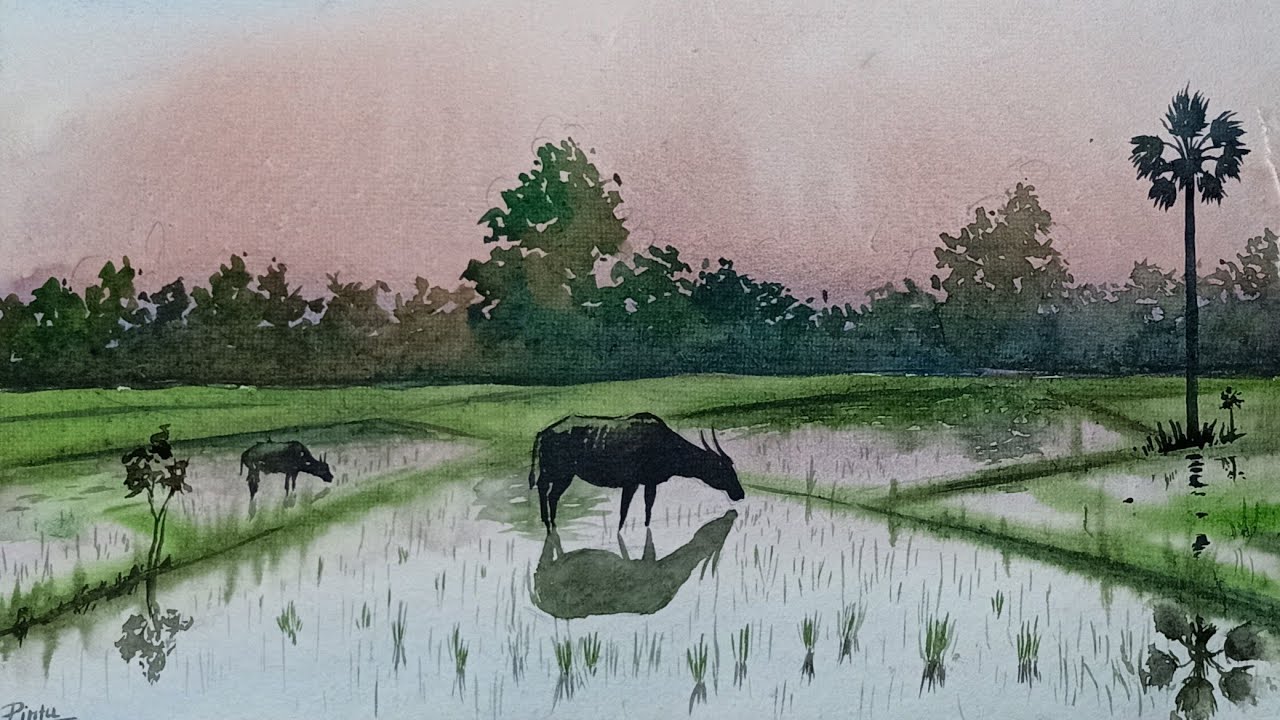A detailed watercolor painting captures a serene wilderness landscape on a textured canvas. The scene features a pinkish-gray sky, creating a somewhat gloomy atmosphere. In the background, a blend of indistinct trees and shrubbery with detached leaves form a green horizon line. 

The landscape below consists of a grassy plain interspersed with three distinct sections of shallow water, resembling a rice field layout: a rectangle on the left, diamond-shaped section in the middle, and a square on the right, each separated by narrow strips of grass. Thin blades of grass emerge sporadically from the water, enhancing the natural feel of the habitat.

Dominating the scene are two cow-like animals with horns, possibly resembling water buffalo, their black silhouettes reflecting in the tranquil water. One animal, larger and nearer, drinks from the central section, while the smaller, more distant one engages in the left section. On the right edge, a tall, silhouetted tree with palm-like fronds adds vertical interest, set against the subtle tones of the twilight sky. This painting's wide aspect ratio further immerses the viewer into its calming, pastoral vibe.